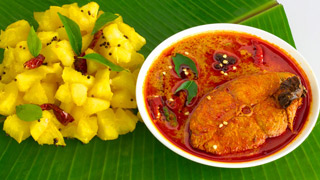This image depicts a close-up view of a vibrant meal displayed on what appears to be a green, plastic placemat. To the left, there is a pile of yellow chunks that resemble pineapple or possibly potato salad. This dish is interspersed with hints of green, likely mint leaves, and possibly some cranberries or other small, red fruits.

On the right side of the image, there is a white bowl containing a rich, red sauce with a piece of meat partially submerged in it. The meat looks tender and might even contain a bone, suggestive of a steak or a hearty cut. The dish is garnished with green herbs, possibly parsley, and includes green and red peppers, hinting at a spicy, flavorful profile. The surrounding liquid is predominantly red but transitions to an orangish-yellow near the top, possibly due to mixed spices or melted cheese.

In the upper right corner of the image, a hint of white, likely the table beneath, peeks through, indicating a close-up, top-down perspective on the food. The combined presentation suggests a hearty, diverse meal served with an emphasis on bright, contrasting colors and rich, savory sauces.